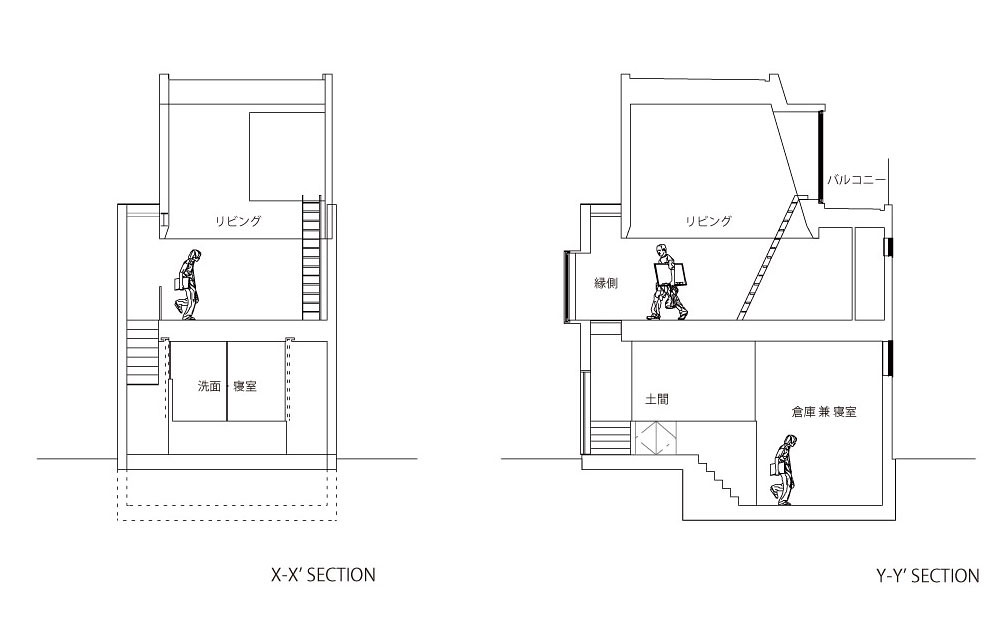The image depicts black and white sketches of building blueprints, divided into two sections labeled as X-X and Y-Y sections. Each section illustrates multiple floors adorned with architectural details, foreign characters, and human figures. In the X-X section on the left, the ground level features two identical window-like squares and a staircase ascending to the first floor, where a person holding a folder walks, approaching a ladder leading to an upper section. In the Y-Y section on the right, the bottom level depicts a person walking while holding papers, with a staircase behind them leading up to the next floor. Here, another person is shown carrying a large white square under their arm, moving towards the left with a ladder leading to the top section. Both sections showcase detailed staircases, ladders, and levels, with foreign characters interspersed throughout, giving an intricate view of a multi-story building in wireframe form.